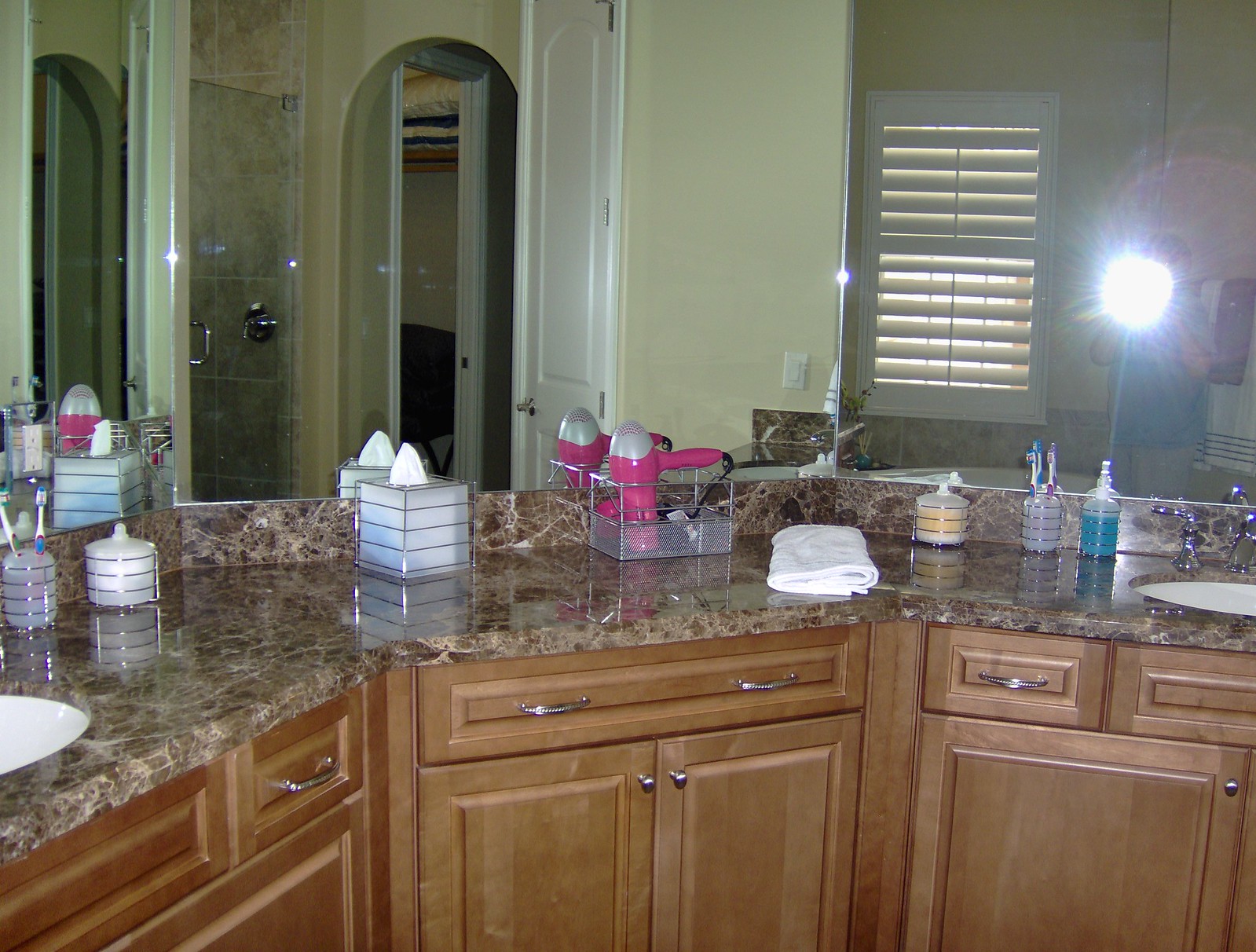This photograph captures an elegant bathroom interior with a sophisticated three-sided beige and brown marble countertop, perfectly fitting into the curved edges of the room. The countertop features two white round basin sinks with sleek silver metal faucets, positioned on the left and right panels, while the center panel remains a solid expanse of marble. 

A slight raised backsplash of the same marble material gracefully edges the sink area, leading up to the upper half of the composition, which is dominated by expansive glass mirrors that reflect various elements of the bathroom.

A variety of neatly arranged items populate the countertop: starting from the left, a toothbrush holder is present next to a closed round holder, presumably containing cotton balls, with a matching frosted glass and horizontal metal wire design. Following, there is a square Kleenex box, a stylish pink and silver hairdryer, a crisply folded white hand towel, another identical round holder filled with a yellow substance, a second toothbrush holder, and a blue bottle of soap, all maintaining a coherent design aesthetic.

The front of the counters, constructed from light brown wood, showcases orderly drawers and cabinets adorned with silver poles and handles, adding to the overall elegance of the space. The mirrors not only amplify the spaciousness but also reflect various facets of the bathroom: a window, an ivory-colored wall, a white door, an arched doorway, and a gray tiled shower, along with a bright white flash from the camera held by the person taking the picture in the rightmost mirror.